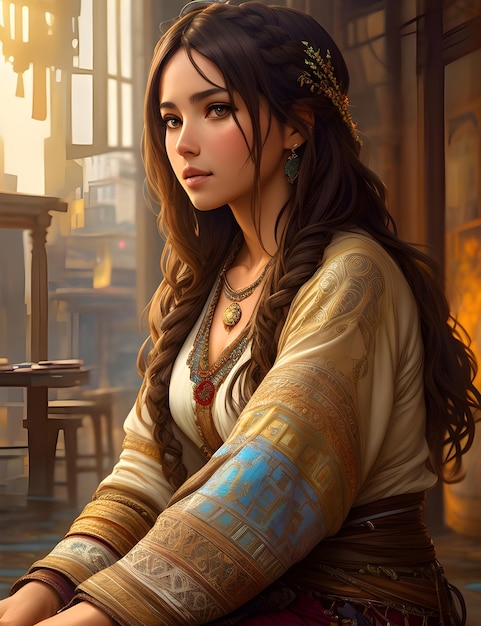The image is a computer-generated artwork of a woman seated in a room with a large window to the front, which allows some light to filter through, softly illuminating the scene. The woman has long, curled dark brown hair that cascades down her back and chest, adorned with gold filaments and a light green hairpin on the left side of her head. Her eyes are a warm brown, and she wears gold earrings set with a green stone on her left ear. She is dressed in an intricately designed robe with a rich array of colors, predominantly featuring blue, gold, cream, and white. The robe has gold patterns along the sleeves and a white center, with a round, red medallion positioned below the collar. Additionally, she wears a gold necklace with a golden round emblem. The room includes a hazy view outside through hanging wooden elements and shows buildings adorned with yellow flags. The overall style of the artwork feels influenced by Indian, Middle Eastern, or possibly Egyptian themes.